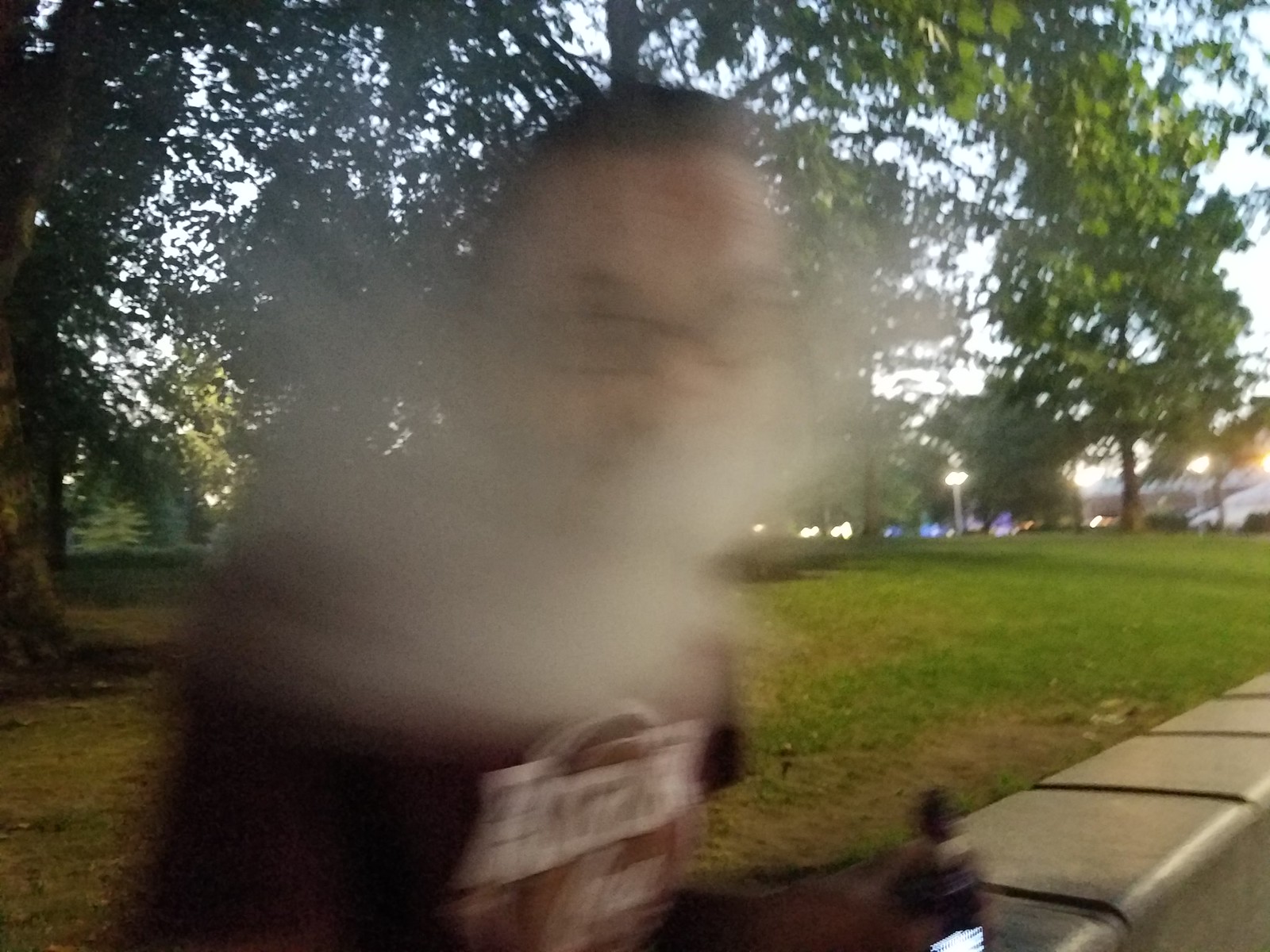This blurred close-up image features a Caucasian individual with dark hair and wearing regular glasses with dark rims. The person appears to be dressed in either a brown or burgundy top that is cut off at the waist, adorned with an emblem on the chest area. The visibility of the person's face is significantly obscured by a white, blurry mark. The background is muted, showcasing what seems to be the person seated on either a chair or a bench. To the right, there is a brown object, possibly part of the seating arrangement. Additionally, a curb, a portion of the street, and a grassy field studded with trees and tiny lights can be seen. Some small buildings are visible in the distance on the right side of the image.